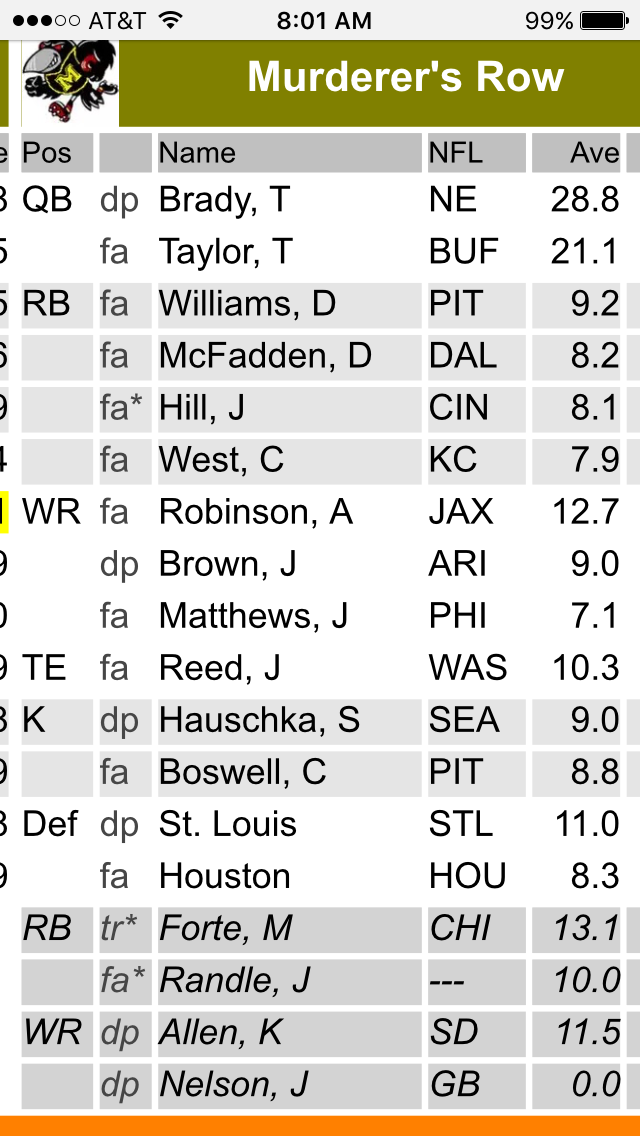This image is a vertical screenshot from a mobile device using AT&T service, captured at 8:01 AM with a 99% battery life. At the top, there’s a thin gray bar indicating the cellular and battery status. Directly below is a green banner with the text "Murderer's Row" in white font, alongside an icon of a cartoon bird wearing a jersey with a large yellow "M". The bird appears to have a gray beak and black feathers and is depicted holding a football. The main portion of the image features a detailed chart with various statistics related to NFL football players. The categories on the chart include "Pause," "Name," "NFL," and "AVE," and it lists several player positions such as QB (Quarterback), RB (Running Back), and indicates their teams and average performance statistics. For example, it mentions "QB, DP, Brady, T., NFL, NE, AVE, 28.8" and "RB, FA, Williams, D., PIT, AVE, 9.2," among others. The stats board continues with numerous entries, highlighting different football players, their positions, teams, and average points, culminating with an orange line at the bottom of the image.